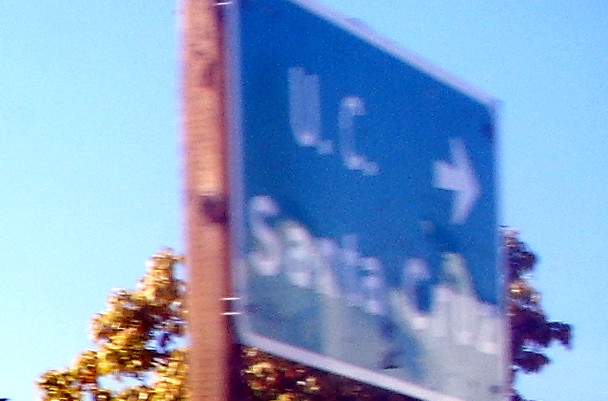A slightly blurred photograph captures a roadside scene, likely shot from a moving vehicle. The focal point is a green road sign with a thin white border, mounted on two dark brown wooden poles. The sign features white lettering stating "U.C." with an arrow pointing to the right, followed by "Santa Cruz" beneath it. The background showcases a tree with foliage in shades of brown and gold, suggesting it might be autumn. Beyond the tree, the sky stretches out in a vibrant blue, adding a serene backdrop to the composition. An indistinct reflection on the sign suggests light interference, contributing to the image's overall blur.